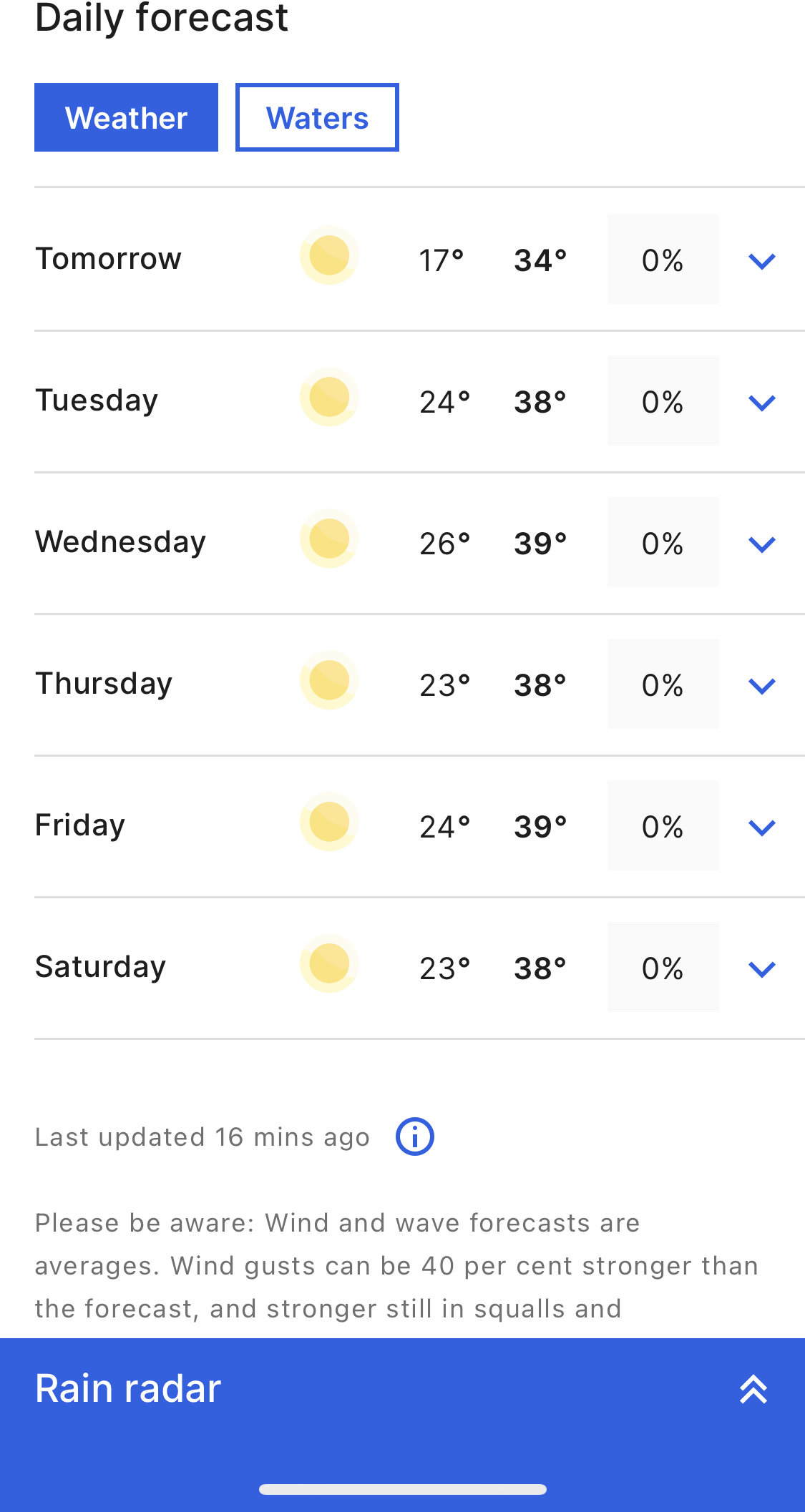The image depicts a mobile device displaying a weather app with a clean white background. At the very top of the screen, in bold black text, it reads "Daily Forecast." Below this header, there are two tabs: "Weather," highlighted in blue with white text, and "Waters," which is highlighted in white with blue text. The "Weather" tab is currently active.

The main section shows the weather forecast for the upcoming days, starting with "Tomorrow," which indicates a low temperature of 17°C and a high of 34°C, with a 0% chance of rain. The forecast for the following days continues in a similar pattern, each indicating sunny weather:

- **Tuesday**: Low 24°C, High 38°C
- **Wednesday**: Low 26°C, High 39°C
- **Thursday**: Low 23°C, High 38°C
- **Friday**: Low 24°C, High 39°C
- **Saturday**: Low 23°C, High 38°C

At the bottom of the screen, it notes that the forecast was last updated 16 minutes ago. There is also a blue box labeled "Rain Radar" at the very bottom of the page.